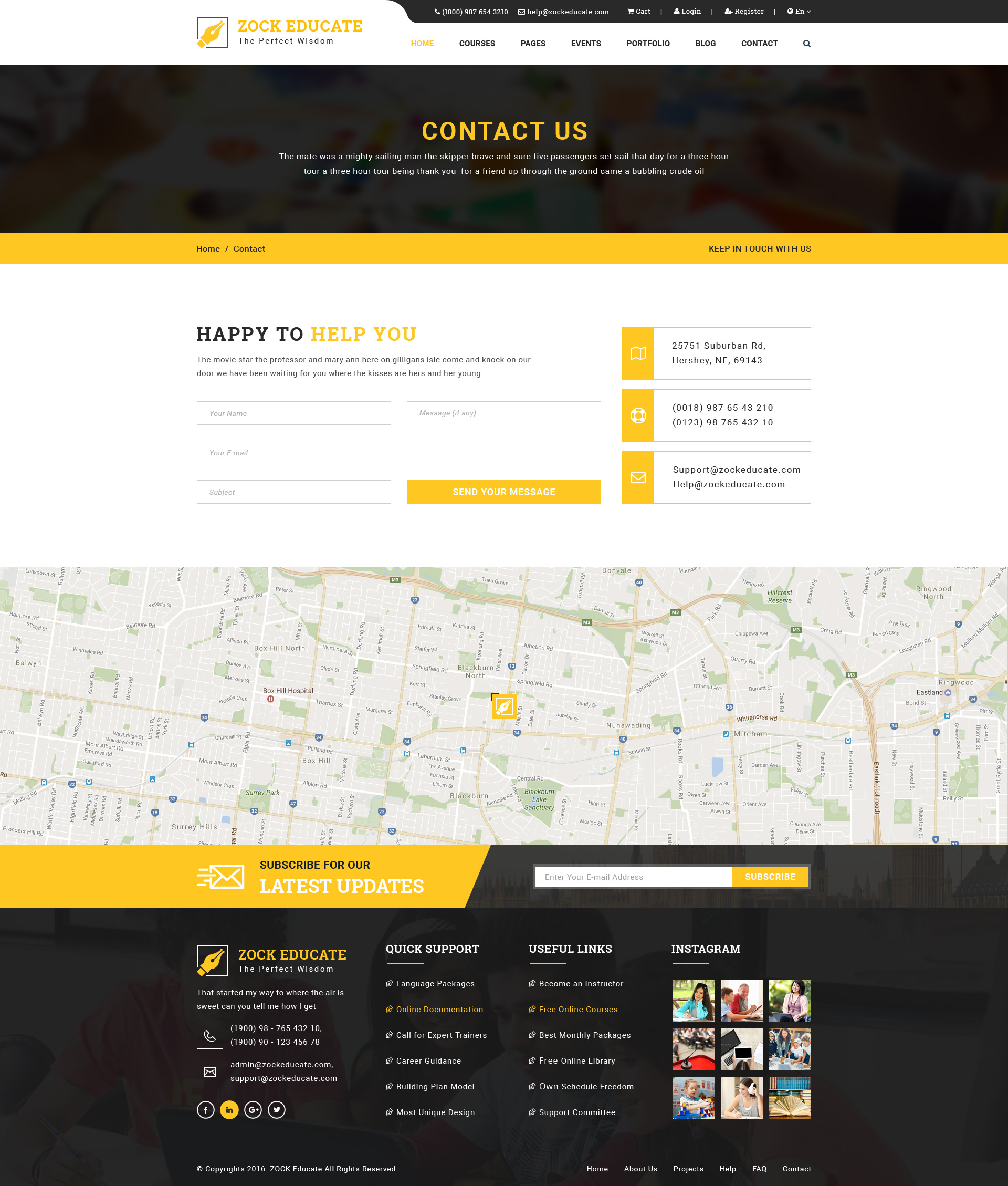This image is a detailed screenshot of the ZocEducate website, branded as "The Perfect Wisdom." The main header features "ZocEducate" in bold yellow text with a logo resembling the tip of a fancy pen with a metal tip. Beneath this is smaller black text that reads "The Perfect Wisdom."

Below the logo, there is a comprehensive menu bar with options including Home, Courses, Pages, Events, Portfolio, Blog, and Contact, along with a search bar. Above this menu bar, a black stripe contains contact details, featuring a phone number (1-800-987-654-23210), an email address, cart, login, register, and language selection icons (showing English).

The primary image below the menu reveals a bold "Contact Us" message in uppercase orange text on a black background. An orange stripe at the bottom of this image features navigation text: Home > Contact, and prompts to "Keep in Touch."

The main section of the webpage is a white background with the heading "Happy to Help You." This section includes three input fields for Name, Email, and Subject, followed by a larger message box. Below these fields is a "Send Your Message" button. On the right, there are three boxes displaying the business address in Hershey, New England, two phone numbers, and two email addresses (Support@ZocEducate and Help@ZocEducate.com).

Further down, a map indicates the business location. Beneath the map, a mostly black section identifies additional resources: Quick Support, Useful Links, and Instagram pages, alongside another phone number and email address. The section also contains a subscribe bar for newsletters or updates and a latest updates section.